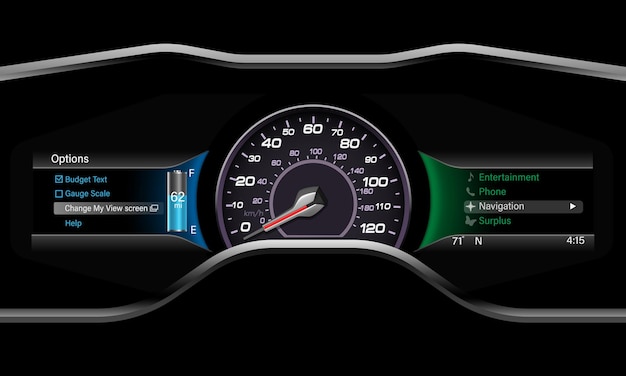The image depicts a detailed car dashboard in a landscape orientation. Central to this dashboard is a dual-scale speedometer with a gray background marked with white and light blue text, indicating speeds in both miles per hour (MPH) and kilometers per hour (KPH); the MPH scale is on the outer ring and the KPH scale on the inner ring. The speedometer ranges from 0 to 120, with white lines demarcating each ten-unit increment. The needle, primarily silver with a red line running through it, points to the speed.

Flanking the speedometer are two digital screens within the black dashboard, which has a slightly wavy silver outline around its edge. To the left, there is a digital options display showing items such as "budget text," "gauge scale," "change my view screen," and "help," all in various text colors. Below this, a fuel gauge indicates '62 miles' to empty, with a partially filled blue bar and white 'F' (full) and 'E' (empty) indicators. 

On the right side, a touch-screen interface provides access to functions such as "phone," "entertainment," "navigation," and "surplus." The screen shows additional information including a temperature reading of '71 degrees' and coordinates or another number in white text. The entire design combines both analog and digital elements, blending traditional dial mechanisms with modern digital interfaces.